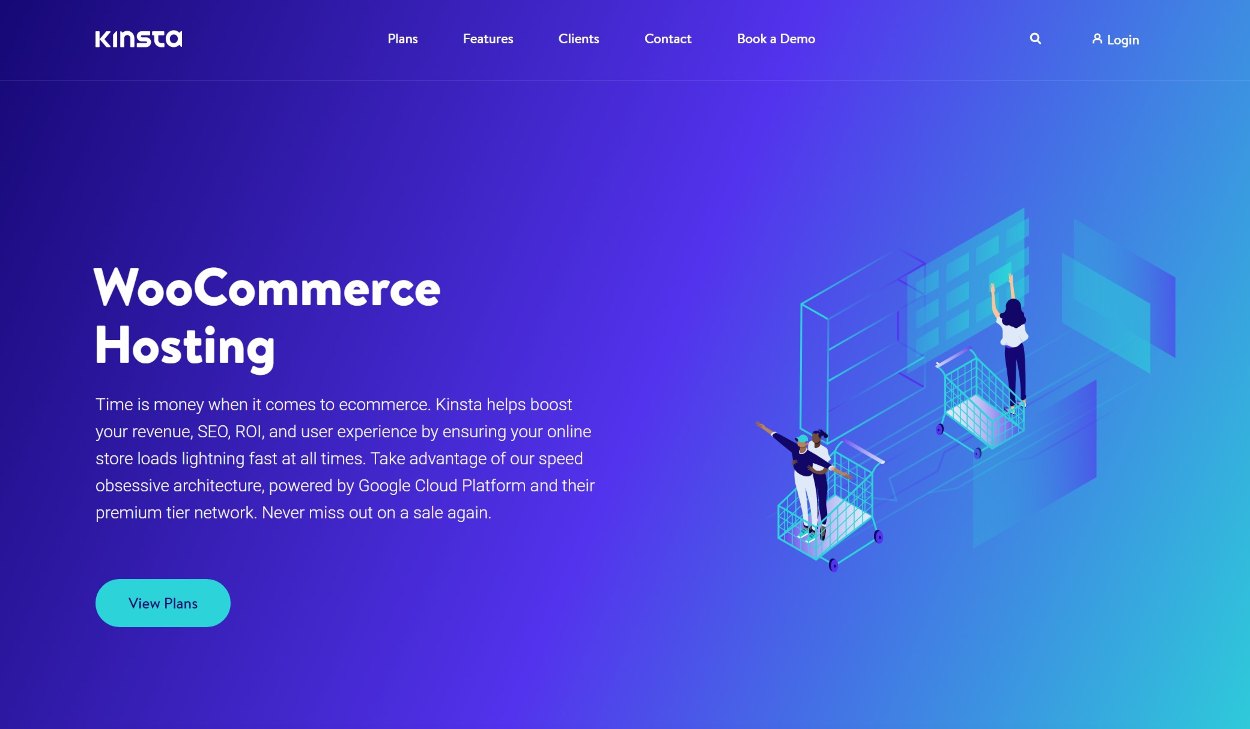The home page of Kinsta WooCommerce Hosting features a striking gradient background, transitioning smoothly from a darker cobalt blue on the left, through a purplish blue, and finally into an almost light sky blue on the right. 

At the top, the header text is displayed prominently in white. From left to right, it starts with "Kinsta" in bold in the upper left corner, followed by navigation links— "Plans," "Features," "Clients," "Contract," and "Book a Demo." To the far right, there's a magnifying glass icon and an icon representing a person, indicating a login option.

Just beneath this header, a thin light line stretches across the page. Centered below it, "WooCommerce Hosting" is boldly presented in large white text. Below this title, a smaller text block reads: "Time is money when it comes to e-commerce. Kinsta helps boost your revenue, SEO, ROI, and user experience by ensuring your online store loads lightning-fast at all times. Take advantage of our speed-obsessive architecture powered by Google Cloud Platform and their premium tier network. Never miss out on a sale again." 

Further down, a light blue oval button invites users to "View Plans" in blue text. To the right of this call-to-action, two shopping cart icons are depicted. One cart contains two people, while a woman stands behind the other cart, reaching for an item on the wall.